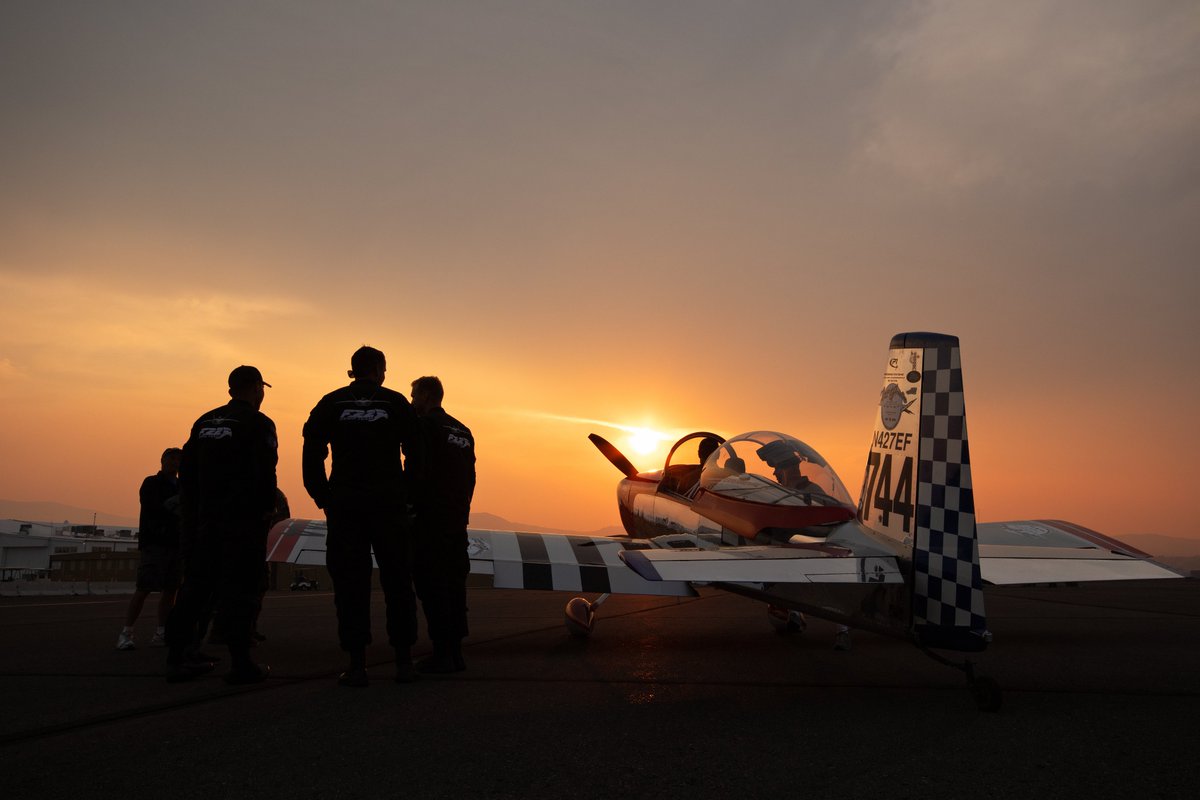In the picture, the sun is setting, casting a gray to orange and purple gradient across the sky. The sun, a dim yellow, peeks through some clouds, adding a soft glow to the scene. In the foreground, there's a plane showing a distinctive black and white checkerboard pattern on its tail and rear wings. It bears the markings "744N" and "W427EF" on the tail, with the letters fading into the background. The plane has a clear glass bubble over the cockpit and appears to be either gray or red in color. On the left side of the image, four men are standing; three of them wear coveralls and hats, with unreadable text on the back of their coveralls. The fourth man, in front of them, is dressed in shorts and tennis shoes, arms folded over his chest. The ground beneath them is a dull gray, complementing the overall twilight ambiance.